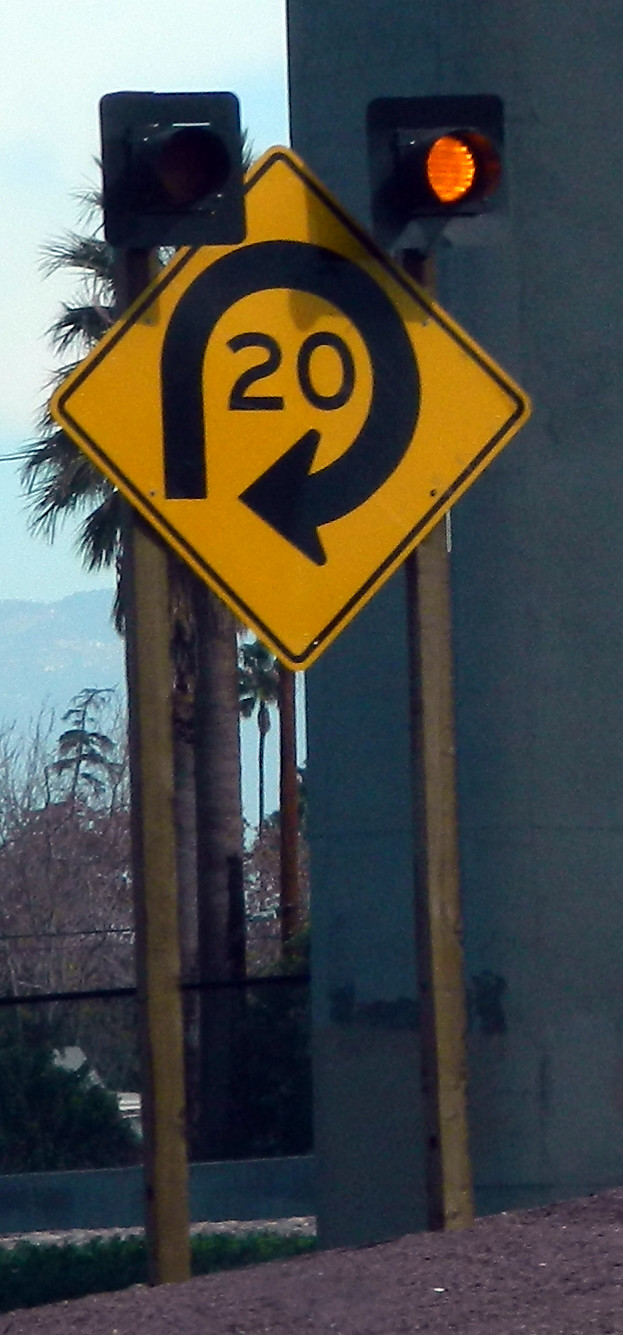The image captures an outdoor scene with a complex interplay of natural and man-made elements. The background showcases a gradient sky transitioning from light to dark blue, descending into a range of hazy hills or mountains. Nestled within this backdrop is a wooded area punctuated with tall palm trees. In the foreground on the right, there's a gray building partially obscured by the scene. A short concrete wall runs across the building's base, extending towards the viewer.

Prominently featured is a street sign held up by two wooden poles. The sign itself is a yellow diamond-shaped warning sign, trimmed with a thin black line. It prominently displays a black, nearly circular arrow that curves into almost a complete loop, ending near a "20" in the center of the sign. The yellow diamond sign is positioned at the midpoint between the poles, which also support two mounted traffic signals. The signal on the right is illuminated with a yellow light, while the left signal is currently unlit.

Below the sign, the ground appears gravelly or could be painted red cement, adding an additional texture to the scene. Stretching between the palm trees and the sign, there seems to be a chain-link fence atop the concrete wall, further enriching the detailed landscape captured in the photograph.